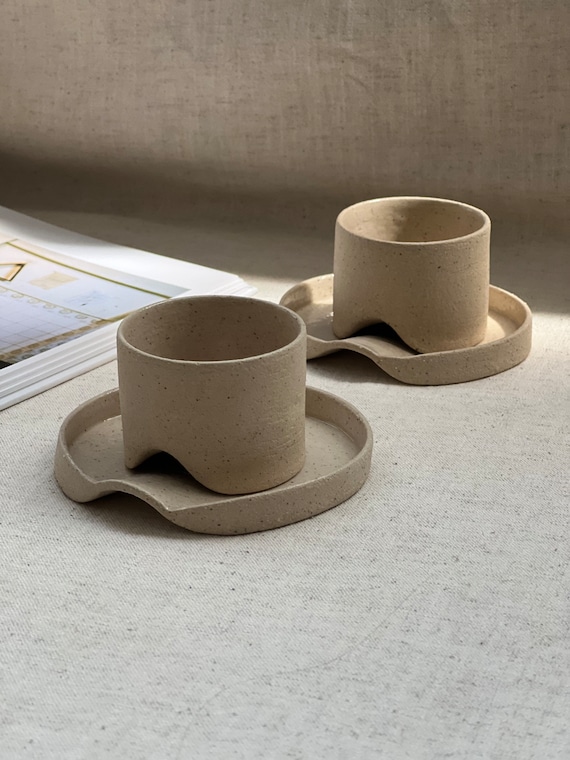This photograph captures two uniquely shaped, beige ceramic cups positioned on matching saucers. Both the cups and saucers are cylindrical with distinctive arched indentations at their bases, elevating them slightly off the surface. The entire setup rests on a light beige, textured cloth that extends upward, serving as both the table and backdrop. To the left of the cups and saucers, there is an open book with a predominantly white cover featuring light blue and gold designs, though the exact details of the image are unclear. The neutral, earthy tones of the scene, coupled with the handcrafted appearance of the ceramics, evoke a subdued and artistic ambiance.